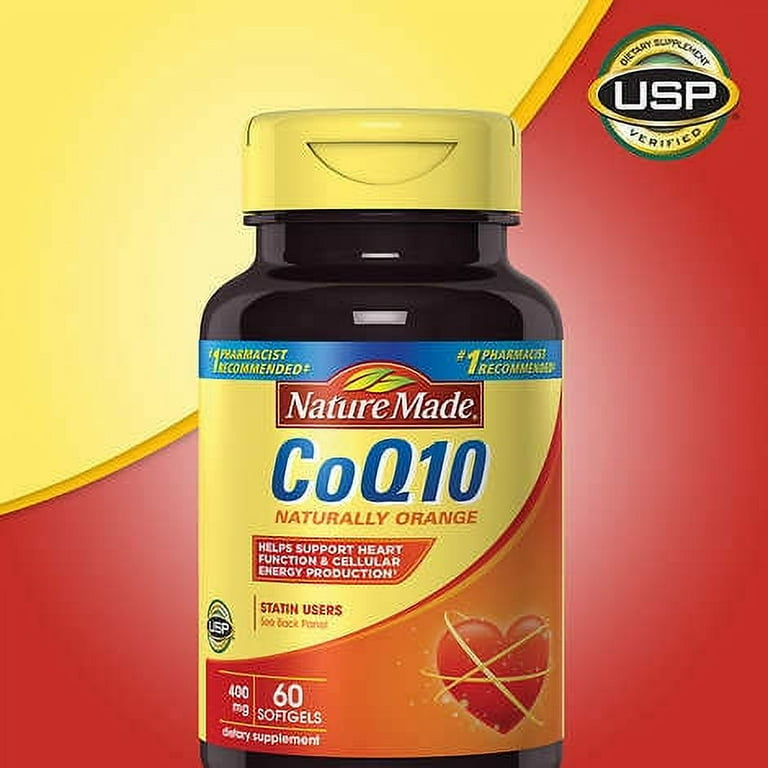The image is an up-close advertisement for a dietary supplement made by Nature Made. The background features a half-cut yellow circle in the top left and yellow and red colors spanning from top to bottom. A green circle in the top right corner reads "Dietary Supplement Verified, USP" with a black oval inside stating "USP". At the center of the image is the product, a translucent dark brown pill bottle with a yellow cap. The label at the top displays "Nature Made" followed by a blue band that reads "Number 1 Pharmacist Recommended" twice. Below that, the label says "CoQ10 Naturally Orange" and highlights its benefits for heart function and cellular energy production. The bottle contains 60 soft gels, each 400 mg, and notes for statin users to see the back panel. Additionally, the bottom right of the label features a red heart emblem wrapped with three gold bands, indicating good health.